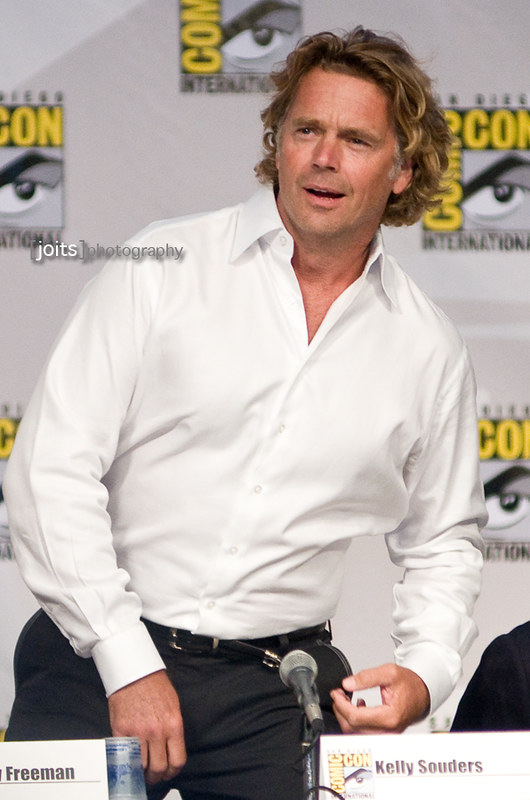The image is a high-resolution photograph taken indoors featuring a white man, likely in his forties, with longer hair that extends past his ears. He is wearing a white button-down shirt with no undershirt, black pants, and a black belt. Positioned in front of a microphone stand, he appears to be standing, slightly tilted to his left while looking towards his right. The backdrop behind him is predominantly white, displaying the Comic-Con International logo adorned with iconography that includes a stylized eyeball graphic.

In terms of background details, there is a watermark that reads "JOITS Photography" above the man's right shoulder. The setting includes two name tags visible at the bottom of the image, one tagged "Freeman" in the lower left-hand corner and the other tagged "Kelly Souders" in the lower right-hand corner. Additionally, the shoulder of another individual is partially visible in the lower right-hand corner, suggesting the presence of a panel or a group setting.

In summary, the image captures a man in business-casual attire at a Comic-Con event, poised ready to speak or engage, with notable textual elements and a professional watermark indicating the photographer.